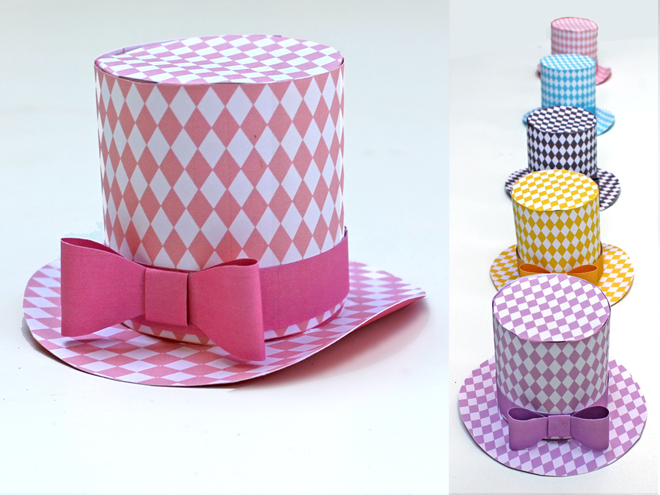This image is a digital advertisement for a series of top hats, featuring a clean, white background and divided into two sections. On the left side, there is a single, prominent top hat with a tall, cylindrical shape and a wide brim. The hat is adorned with interlocking pink and white diamond patterns and is accented with a pink ribbon around its base.

The right side of the image displays a vertical array of five top hats, arranged from top to bottom. Each hat showcases the same interlocking diamond pattern but in different color combinations. From top to bottom, the hats are colored pink and white with a hidden ribbon, blue and white with a blue ribbon, black and white with a black ribbon, yellow and white with a yellow ribbon, and purple and white with a purple ribbon. Each hat's ribbon color matches the corresponding primary color of the hat, but some ribbons are obscured by overlapping hats in the arrangement.